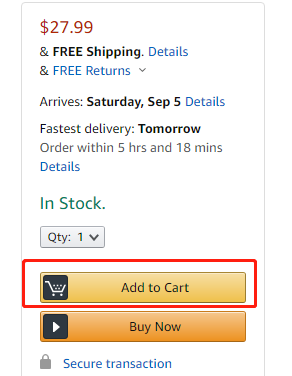The image displays a screen from Amazon's shopping website. At the top left corner, the price is prominently shown in red, marked as $27.99. Below this, the text "Free Shipping" is displayed, also in red. Next to it, a blue "Details" button allows users to click for additional information, which likely pertains to any stipulations regarding the free shipping offer. Moreover, there's another blue link indicating "Free Returns," with a dropdown menu for more details.

The expected delivery date is also presented; in bold letters, it states "Arrives Saturday, September 5th" with a link for further details. An option for expedited shipping is available, promising the fastest delivery by tomorrow, provided the order is placed within the next five hours and eighteen minutes, as specified in bold. Another detail link is situated beneath this information.

Indicating availability, the text "In Stock" is written in green. The quantity box, initially set to one, can be adjusted via a dropdown menu. Users have the option to either "Add to Cart" or "Buy Now," with both buttons highlighted in an orangish-red hue. Currently, the "Add to Cart" button is bordered in red, signifying its active state. Below these buttons, there is an icon of a lock accompanied by the text "Secure transaction," emphasizing the safety of the purchase. 

The entire interface is enclosed within a defined box, with the color scheme predominantly featuring red for pricing and important highlights, blue for additional details and return options, and orangish-red for action buttons.